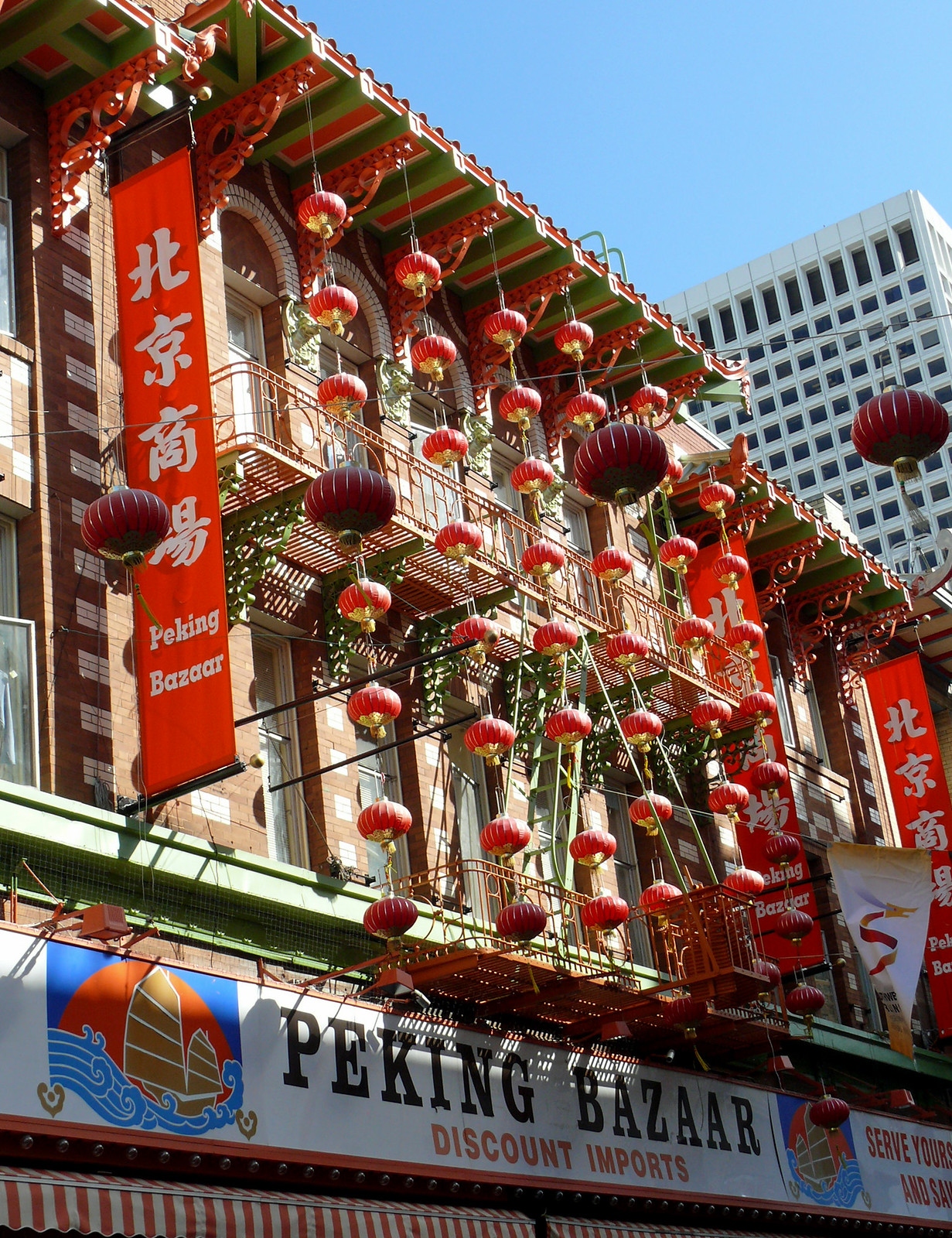This photograph captures the exterior of a building that houses the Peking Bazaar, adorned with vibrant decorations. There are numerous, festively hanging red and gold Chinese paper lanterns strung vertically along the roofline, creating a cascading pattern. Prominently displayed is a large white banner with red roofs and blue wave caricatures above the store entrance, proclaiming "Peking Bazaar Discount Imports." Flanking the building on either side are tall vertical red banners with white Chinese lettering also stating "Peking Bazaar." The building features two stories of windows above the main banner. To the upper right of the image, a clear, cloudless blue sky frames the scene, with the edge of a towering white skyscraper visible in the background, suggesting an urban setting. The overall composition, along with the lanterns and banners, evokes a festive atmosphere typical of a Chinatown in a U.S. city, despite the reference to historical Peking.